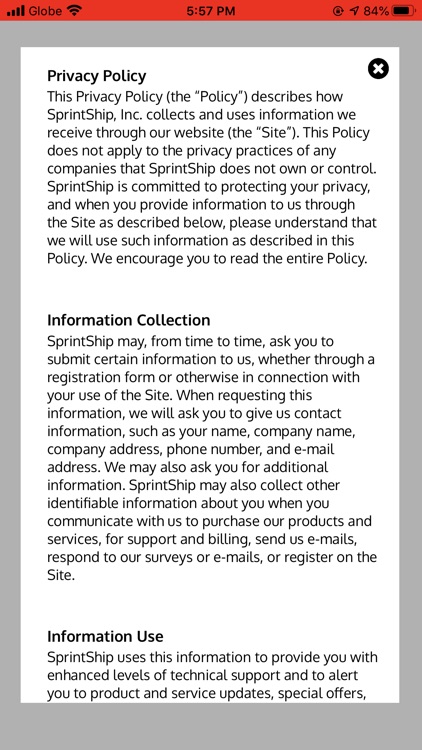Detailed Caption:

The image displays a black text on a white background detailing Sprint Ship Inc.'s Privacy Policy. At the top, it prominently states "Privacy Policy." The policy outlines how Sprint Ship Inc. collects and uses information gathered through their website. It clarifies that this policy does not cover the privacy practices of companies not owned or controlled by Sprint Ship. The company emphasizes its commitment to protecting users' privacy and insists on using the provided information only as described in the policy. Users are encouraged to read the entire document.

The policy section titled "Information Collection" mentions that Sprint Ship may request personal details, including name, company name, company address, phone number, and email address through registration forms or other interactions on the website. It might also collect additional identifiable information when users communicate with them for purchases, support, billing, through emails, surveys, or registrations.

The "Information Use" section explains that the collected data enables Sprint Ship to offer enhanced technical support and inform users about product updates and special offers.